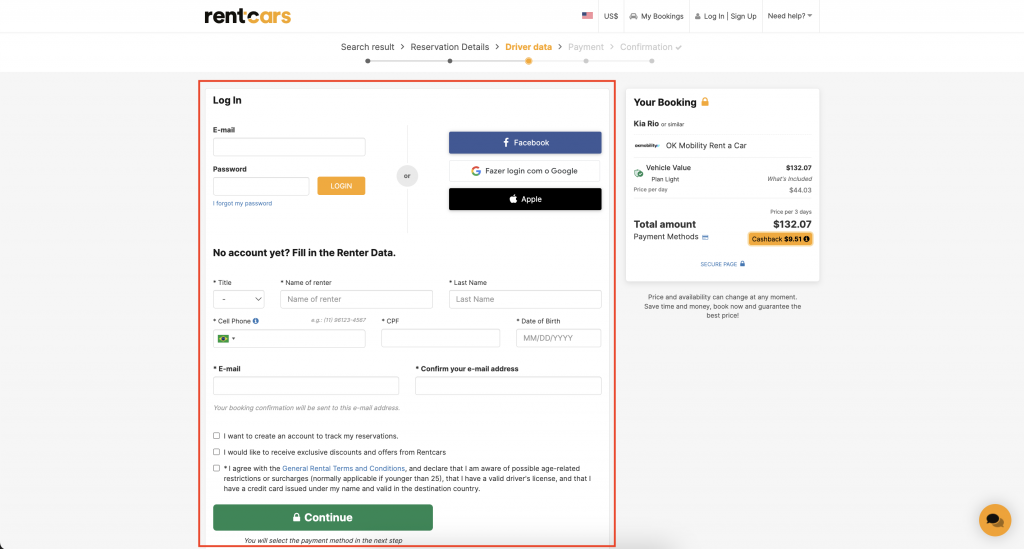The image depicts a landing page for a car rental service. At the top of the page, the heading "Rent Cars" is prominently displayed in black and orange colors. Directly below this heading, several sections are listed: "Search Results," "Reservation Details," and "Driver Data."

On the right side of the screen, there are additional links: "My Bookings," "Login," "Sign Up," and "Need Help," indicating various user options and support features.

Underneath the "Rent Cars" heading, there is a login form. The form includes fields for "Email" and "Password," as well as options to log in via "Facebook," "Google," and "Apple." For new users, a prompt reads, "No account yet? Fill in the renter data."

The sign-up section requests detailed personal information, including "Title," "Name of Renter," "Last Name," "Cell Phone," "Email," "Date of Birth," and a field to "Confirm Your Email Address." Below these fields, there are checkboxes allowing users to opt-in for tracking their reservations and receiving discounts and offers. Users must also agree to the "General Rental Terms and Conditions" before proceeding.

At the bottom of this form, a green button labeled "Continue" can be seen. Additionally, a smaller pop-up window on the right side of the screen provides a summary of the user's current booking, displaying "Vehicle Value" and "Total Amount."